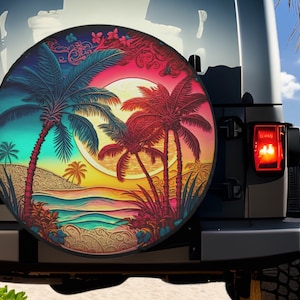The image depicts a close-up of the back of a gray Jeep, though it's unclear whether the image is a photograph or a digital mock-up due to the high level of detail and close cropping. The right tail light is illuminated, adding a touch of realism. The main focus is the spare tire cover, which features a vivid, customized design. The artwork on the cover showcases a tropical beach scene, with palm trees partially obscuring a moon or sun. The scene is divided into contrasting colors: pinks and reds dominate the right side, while blues and yellows highlight the left, creating a visually striking effect. The sandy beach at the bottom of the cover is rendered in light brown or off-white tones. Limited to just one visible wheel and the back end of the Jeep, the image offers a snapshot, rather than a full view, of the vehicle. The overall effect is a detailed and colorful depiction of a serene desert oasis.